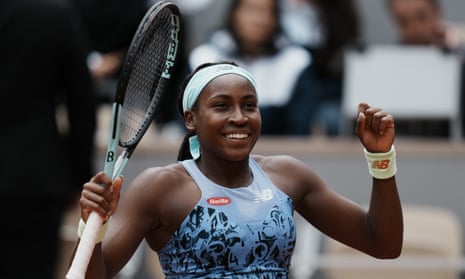This photograph, slightly wider than it is high, captures a chest-up shot of the young American tennis star Coco Gauff. She radiates celebration, likely having just won a match or a significant point. Gauff's dark, somewhat shiny skin is highlighted at her shoulders, emphasizing her athletic build and visible muscles. She wears a light blue tank top adorned with dark blue designs and commercial logos, including a red symbol with white letters and the "NB" logo of New Balance.

Coco's right hand, sporting a white wristband with the red "NB" logo, holds her tennis racket high, showcasing its white handle with green and black accents on the metal frame. Her left arm is bent, and her fist is clenched in a triumphant gesture. A light greenish-blue headband secures her hair as she beams a broad, victorious smile.

The background of the image is blurred, but two judges can be vaguely seen: a female judge placed directly above Gauff, and a male judge to her right, seated, perhaps in front of a laptop. The upper-left corner falls into shadow and focus fades away. This spirited snapshot perfectly encapsulates the exuberance and determination of Coco Gauff at a triumphant moment in her tennis career.